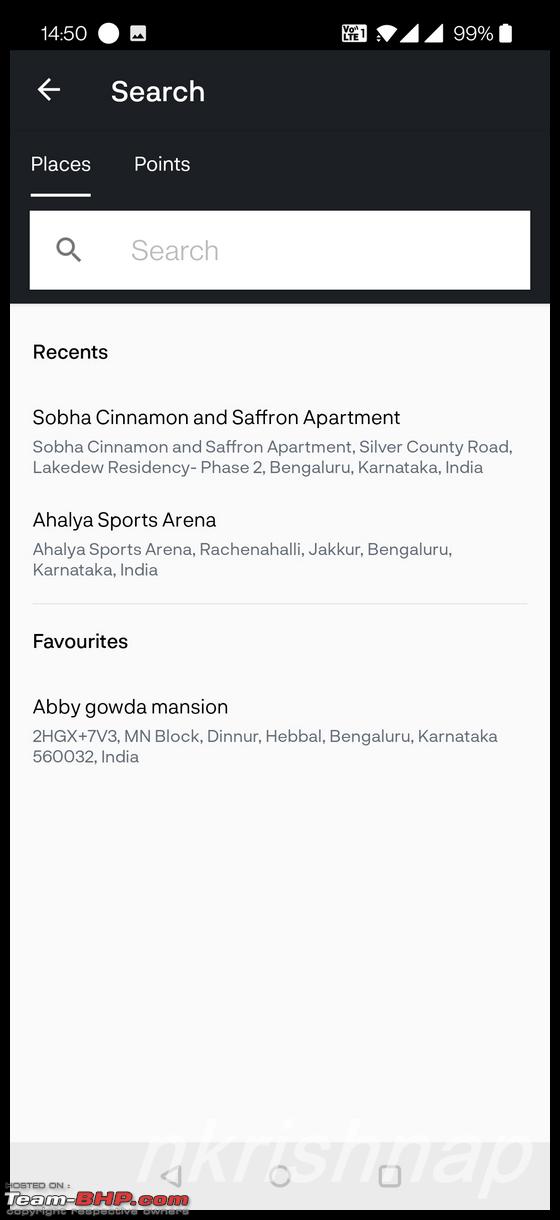The image features a series of graphical elements and text, arranged in a structured layout. 

At the top, there is a black rectangle displaying the number "1450." Adjacent to this, there's a white circle, followed by a white square that contains an unidentifiable element. Alongside these, there is a probable QR code, a Wi-Fi symbol, and two triangles. Next to the triangles, the percentage "99%" is displayed, with a battery icon indicating a high charge level.

Below this top section, a gray rectangle with a white left-pointing arrow and the text "Search" are prominently displayed. Underneath, there are subsections labeled "Places" and "Points," with a line underscoring "Places." 

Further down, there's a white search bar with a magnifying glass icon, labeled "Search." Below the search bar, you will find a black-outlined white rectangle with the words "Recents" inside. Listed under "Recents" are "Soba," "Cinnamon," and "Saffron Apartments," followed by additional text too small to decipher, and then "Lay House Sports Arena" with similarly small text beneath it. 

A section titled "Favorites" follows, highlighting "Abby Gounda Mansion" along with more largely unreadable text.

Lastly, at the bottom of the image, a light gray rectangle contains several elements: white text outlined in black, some red text which is difficult to distinguish but seems to include "something dot com," a left-pointing triangle outlined in gray, a circle outlined in gray, and a square also outlined in gray.